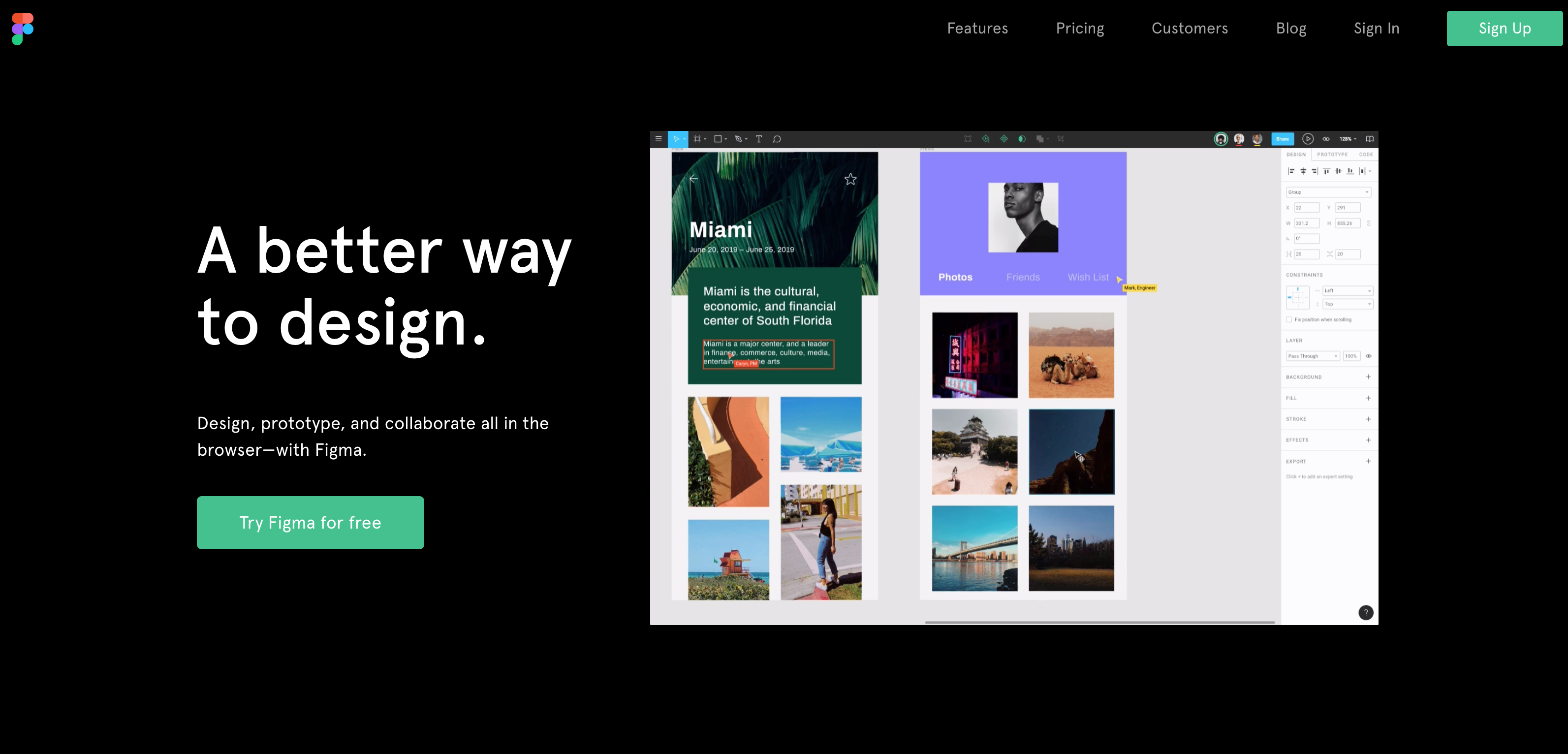**Website Screenshot on Desktop with Figma Branding**

This screenshot captured from a desktop presents a sleek and modern website interface against a black background. In the top-left corner, a vibrant logo comprised of five colored circles is prominently displayed, representing the brand. Adjacent to the logo, the top menu features essential navigation options: **Features**, **Pricing**, **Customers**, **Blog**, and **Sign In**. Completing the header is a distinctive green button labeled **Sign Up**.

The main focal point of the page is the central headline, written in bold white text: "A better way to design". Directly beneath this headline, smaller text elaborates on the message: "Design, prototype, and collaborate all in the browser with Figma". A green button nearby encourages user interaction with the call-to-action: **Try Figma for free**.

On the right side of the page, there is an embedded screenshot that visually demonstrates the use of Figma within the interface. The screenshot showcases various design elements and layouts, including a green leafy background promoting "Miami" and accompanying descriptive text. Another layout is displayed to the right, featuring a purple background and an image of a person, further emphasizing the versatility and creativity enabled by Figma.

Overall, this website encapsulates a smooth user experience, guiding visitors through its features with clear visual aids and interactive elements.